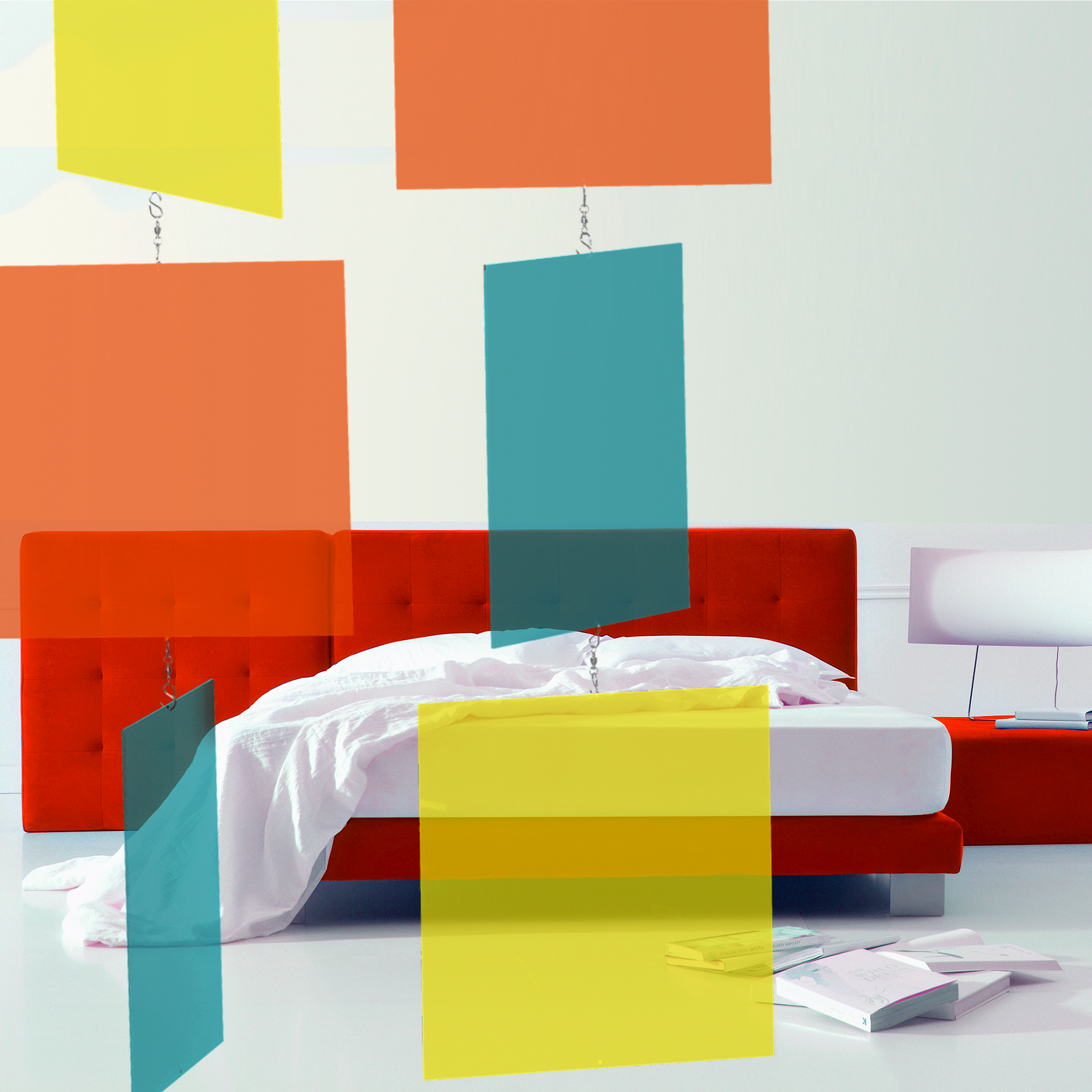This image depicts a modern bedroom adorned with a red padded headboard and a matching red bed frame. The bed is outfitted with white fitted sheets, a white top cover that drapes partially onto the white floor, and white pillows. One of the bed's legs is notably gray. Adjacent to the bed stands a red side table, bearing a white lamp with a rectangular shade and a small stack of books. Scattered across the floor in front of the bed are several books and magazines.

The room's wall is also white, serving as a backdrop to two hanging chains of semi-transparent squares that add a splash of color to the scene. The first chain features a yellow square, an orange square, and a teal square, while the second chain consists of an orange square on top, followed by a teal square, and a yellow square. These vibrant panels create a cheerful atmosphere, accentuating the room's modern decor.